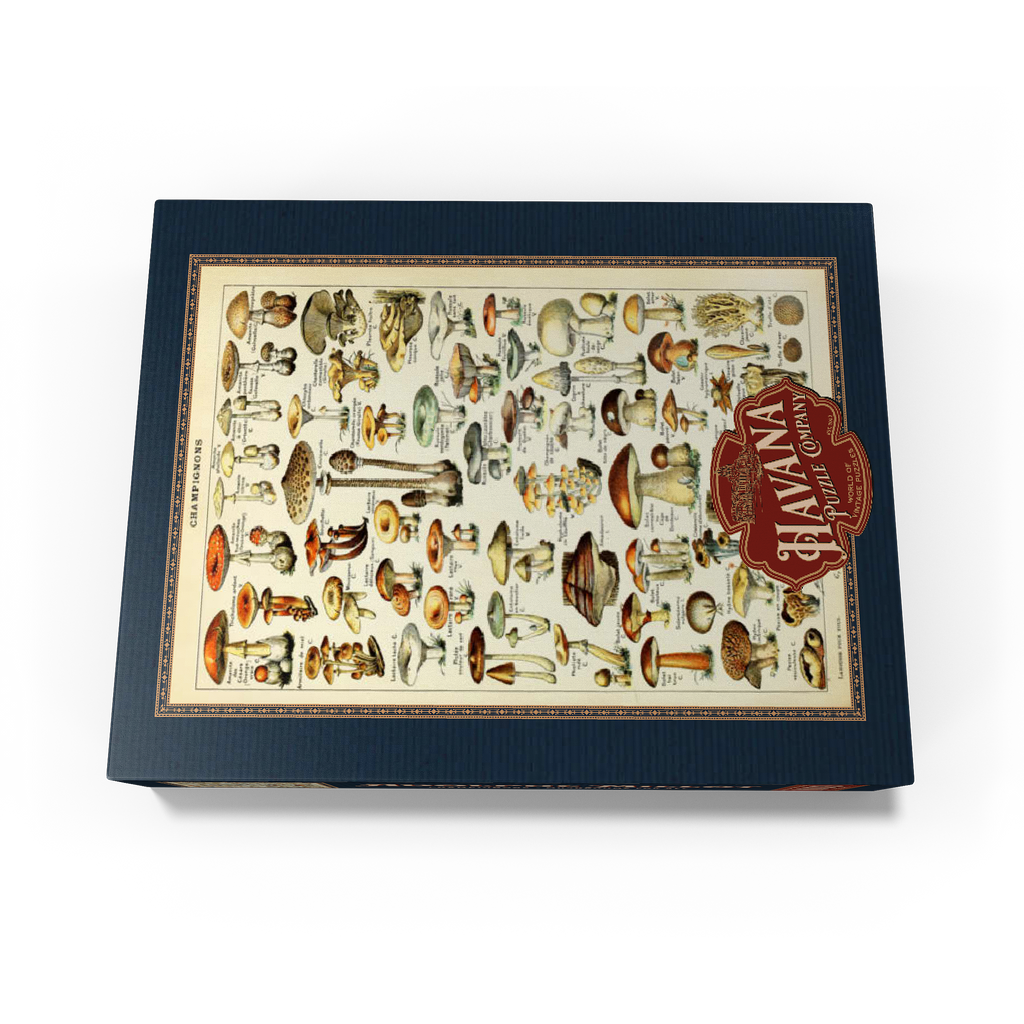The image depicts a detailed poster, likely printed by Havana Puzzle Company, featuring an array of mushroom illustrations against a dark blue background. The poster, which measures approximately 8x12 or 10x13 inches and appears to be rotated 90 degrees in the picture, showcases an extensive collection of colorful mushrooms. Each mushroom is meticulously illustrated and labeled with its name and additional information in very tiny font. The top of the poster prominently displays the word "Champignons" in small text. The poster's design includes rows and rows of mushrooms in various shades—orange, white, brown, and yellow—some even spotted, reflecting a rich diversity in fungi. At the bottom of the poster, a red logo with white text indicates "Havana Puzzle Company," although there is more writing that is too small to decipher. The entire piece not only serves as a botanical illustration but also hints at its connection to puzzles, appealing to both mushroom enthusiasts and puzzle aficionados alike.